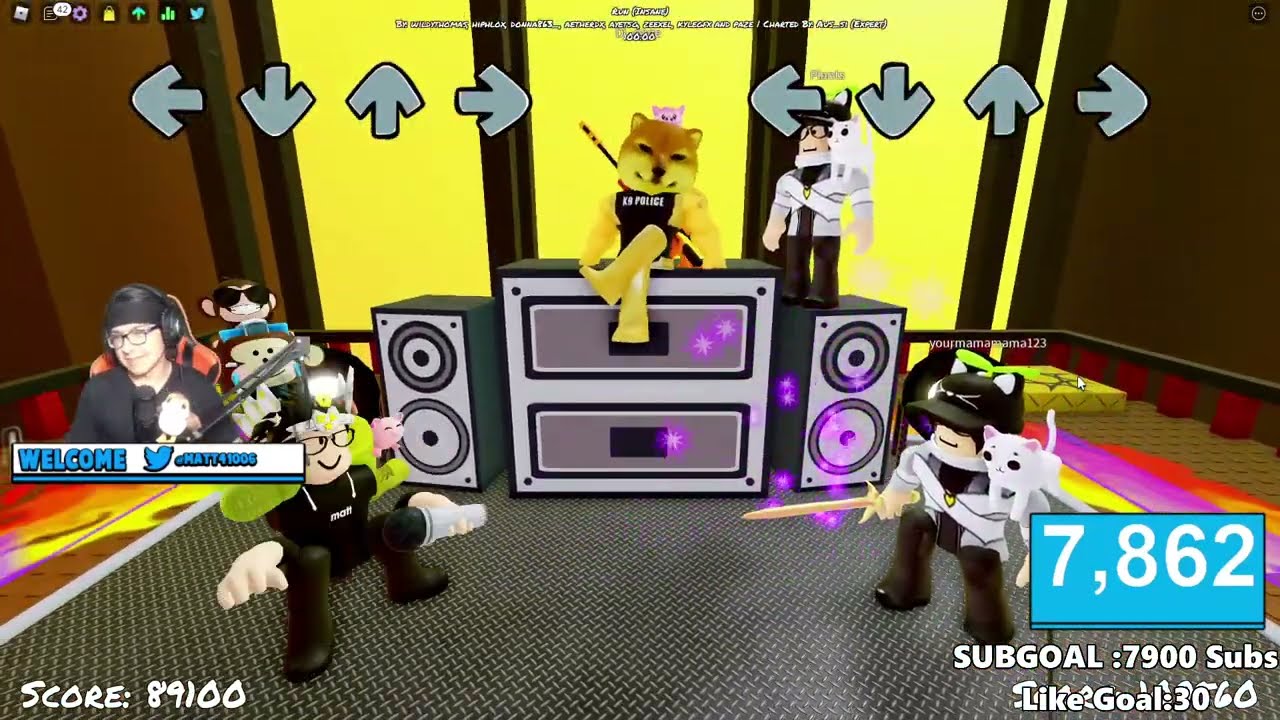The image is a screenshot from a video game showcasing a detailed stage setup with various speakers and characters. At the center of the stage is a prominent square speaker with a black top and sides, featuring gray and black squares with scattered purple dots. On either side of this main speaker, additional speakers with circular fronts and dark black casings surround it. Sitting atop the central speaker is a cartoon character resembling a canine, possibly a Sheba Inu, wearing a vest labeled "Canine Police" and sporting a crossed-leg posture. 

To the right of this speaker, there's an image of another character with a cat perched on its shoulder, facing left. Below, another character with a similar setup—a cat on the shoulder and wielding a sword—also faces left. On the left side of the stage is a picture of a person wearing black glasses, headphones, and a black shirt while speaking into a microphone. Accompanying this image are UI elements such as the text "welcome," the Twitter logo, and a hashtag.

Above the stage, directional arrows (pointing left, right, up, and down) are arranged in sets of four on both the left and the right sides. The bottom left corner of the screenshot displays "score: 89100." The bottom right corner features a blue box with white text reading "7,862." Below that, it lists "sub goal: 7,900 subs" and "like goal: 30."

The back wall of the stage is lined with yellow panels held together by a black frame, while the far left and right walls are brown. The center includes an open section constructed from corrugated steel, adding texture to the stage setup.